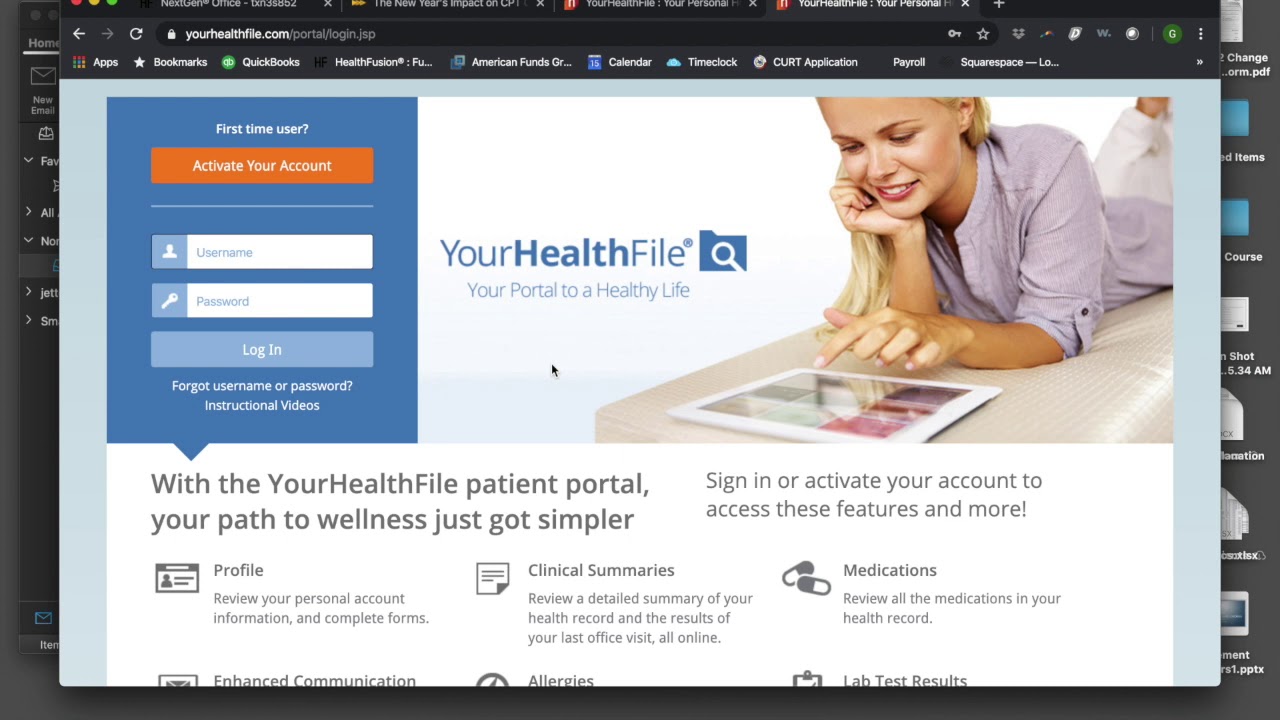A screenshot of a computer desktop showcasing a navigated page from the Your Health File portal. The uppermost tab is highlighted, revealing the portal's main page titled "Your Portal to a Healthy Life." The page prominently features an image of a woman lying on a cushion, smiling with her chin cradled in her right hand while her left hand is poised to touch the screen of a white tablet in front of her. Adjacent to this image is a blue section where new users can activate their accounts, marked by the header "First Time User" in white text. Below this header is an orange and white button labeled "Activate Your Account."

Beneath the activation section, there are two entry fields awaiting user input, the first labeled "Username" and the second "Password," followed by a light blue "Login" button. This is followed by a white window containing enlarged dark gray text that reads "With Your Health File, Patient Portal, Your Path to Wellness Just Got Simpler." Accompanying instructions in smaller text state, "Sign In or Activate Your Account, Access These Features, and More," highlighting features available through the portal such as Profile, Clinical Summaries, Medications, Enhanced Communication, Allergies, and Lab Test Results.

The user's desktop background is dark gray with various colored icons scattered across it.